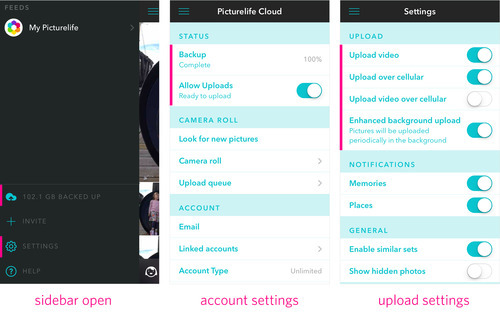**Descriptive Caption:**

The image is a composite of three side-by-side screenshots. 

**Left Screenshot:**
- The background is black.
- Text at the top reads: “My Picture Life.”
- Below it, “102.1 GB backed up.”
- Additional options listed: “Invite,” “Sutton,” “Help.”
- At the bottom, in purple text: “Sidebar Open.”

**Center Screenshot:**
- The header is black, displaying “Picture Life Cloud.”
- Underneath, the background shifts to light blue with the word “Status” written.
- Below it, on a white background with a purple border on the left: “Backup Complete 100%.”
- Additional text reads: “Allow Upgrades, Ready to Upload,” followed by a progress bar oriented to the right.
- Further down, a light blue box labeled “Camera Roll.”
- Below that, a white background with the text: “Look for New Pictures, Camera Roll, Upload Queue.”
- Lastly, another light blue section labeled “Account,” followed by a white background listing: “Email, Listed Account, Account Type.”

**Right Screenshot:**
- Similar thematic elements as the center screenshot, elaborating on the same applications and statuses, providing a cohesive summary of the user's Picture Life application status and available options.